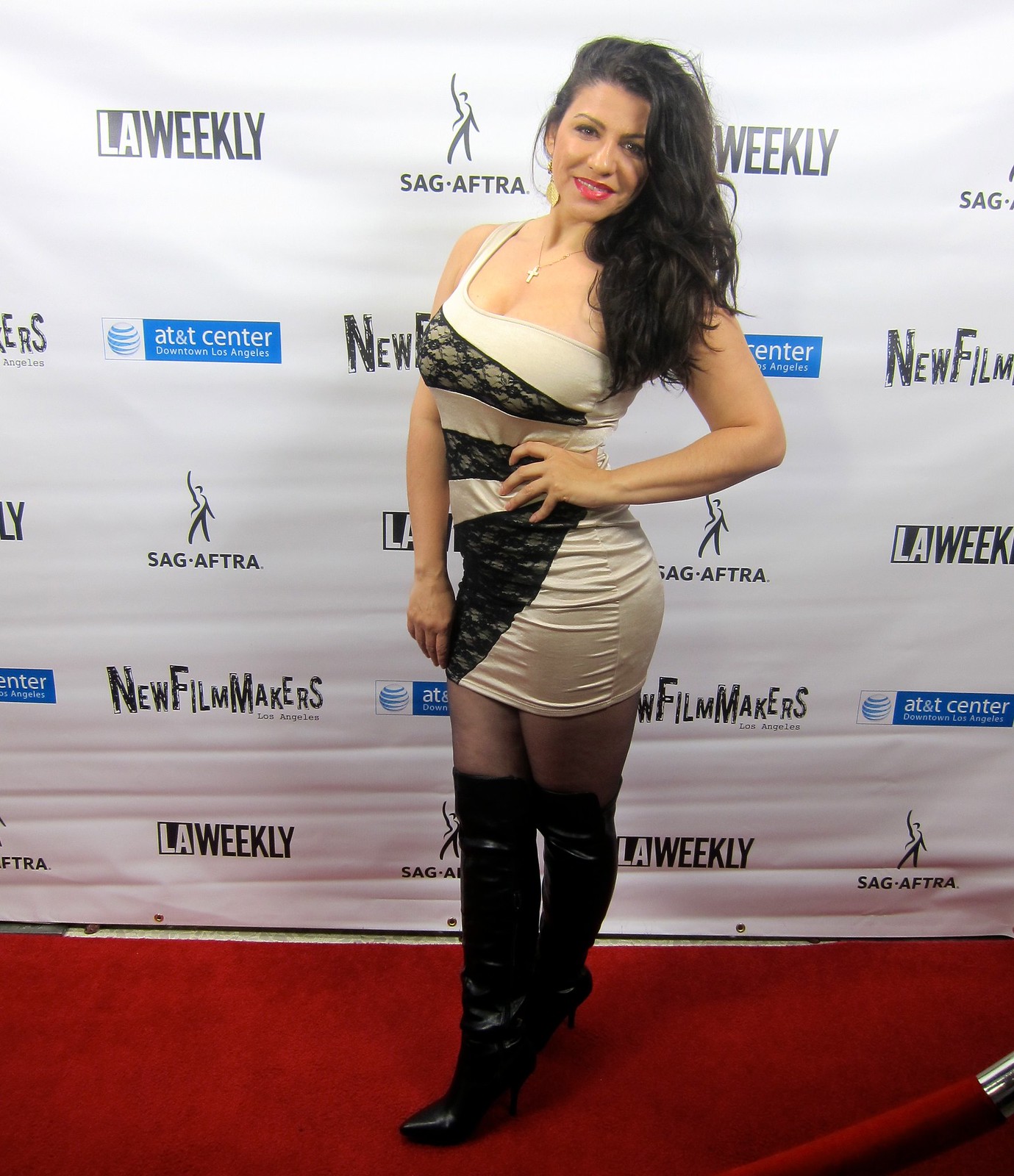In this photograph, a woman is prominently standing on a red carpet at an indoor event, centered in front of a white backdrop adorned with the logos of LA Weekly, SAG-AFTRA, the AT&T Center (logo in blue), and New Filmmakers, indicating the sponsors. With long brown hair elegantly pulled to one side, she gazes directly at the camera, exuding confidence. She is attired in a striking white dress with a black lace accent wrapped around her waist three times, and a necklace with a pendant adding a touch of sophistication. Her ensemble is completed with high-heeled, thigh-high black boots. To her right, a red-and-metal barrier slightly peeks into the frame, suggesting a measure in place to keep the public at bay. The overall scene captures the glamour and exclusivity of what appears to be an awards show or a significant industry event in Downtown Los Angeles.